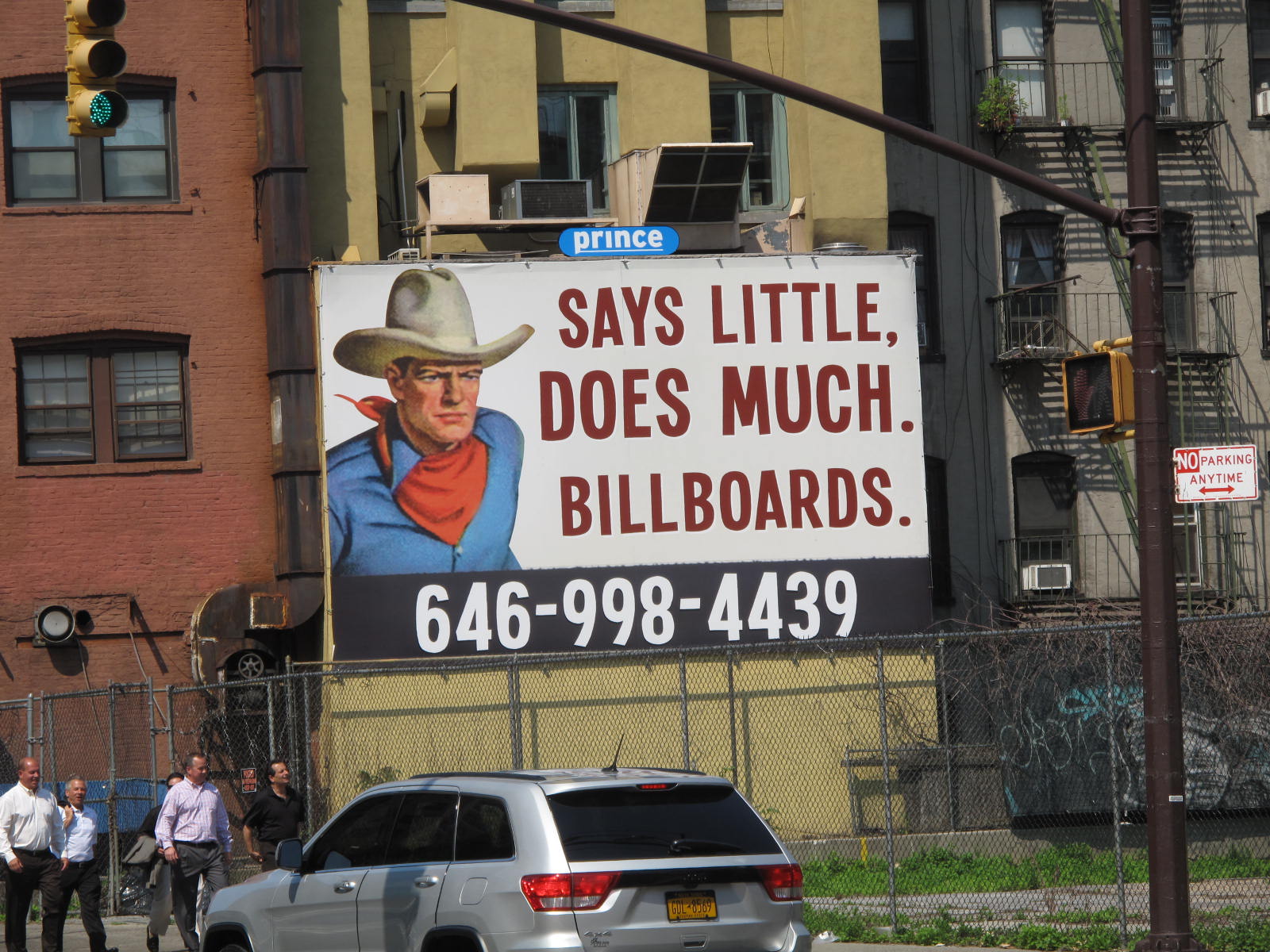Five businessmen, dressed in collared shirts and dress pants, are walking in a group. Behind them, three buildings of distinct colors stand: one dark red, one light yellow, and one medium gray. A prominent billboard featuring the message "Prince Says Little Does Much Billboards" and the phone number 646-998-4439 is visible. The billboard showcases a cowboy in a blue long-sleeve collared shirt, a red bandana tied around his neck and back, and a beige cowboy hat.